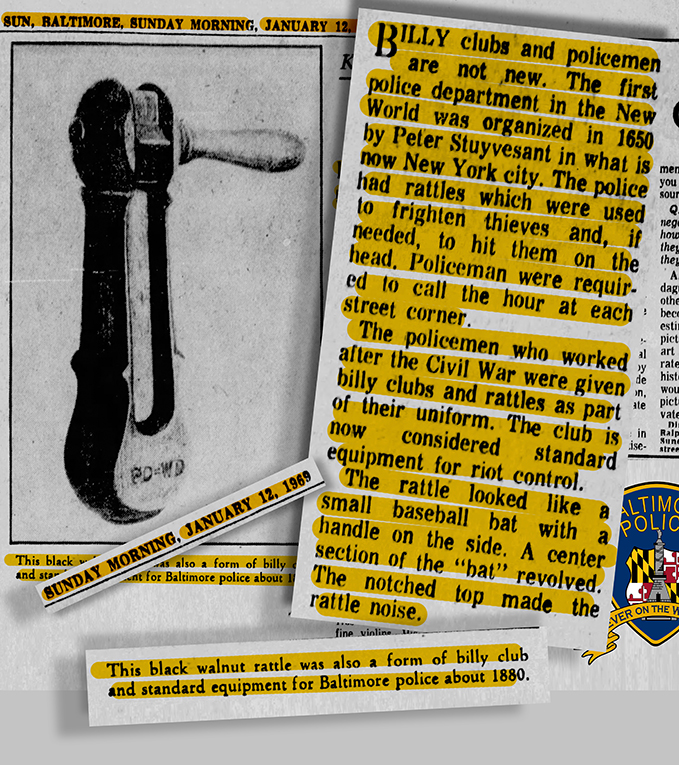This black and white image, seemingly a scan from a January 12, 1969 issue of The Sun Baltimore, features a detailed examination of billy clubs once used by the Baltimore Police. On the left side, underneath a grainy close-up photograph, is the depiction of an old-fashioned billy club, made of wood with a handle that could be spun around, once standard police equipment until about 1880. The right side displays several highlighted texts from the newspaper; the primary article discusses the historical use of billy clubs and rattles by policemen dating back to 1650 in New York City, emphasizing that such tools for subduing suspects are "not new." More text boxes, also highlighted, occupy the lower portion, including references to dates and supplementary context about the billy clubs. In the bottom right corner, partially visible, is the Baltimore Police logo, a police shield adorned with the Baltimore flag.